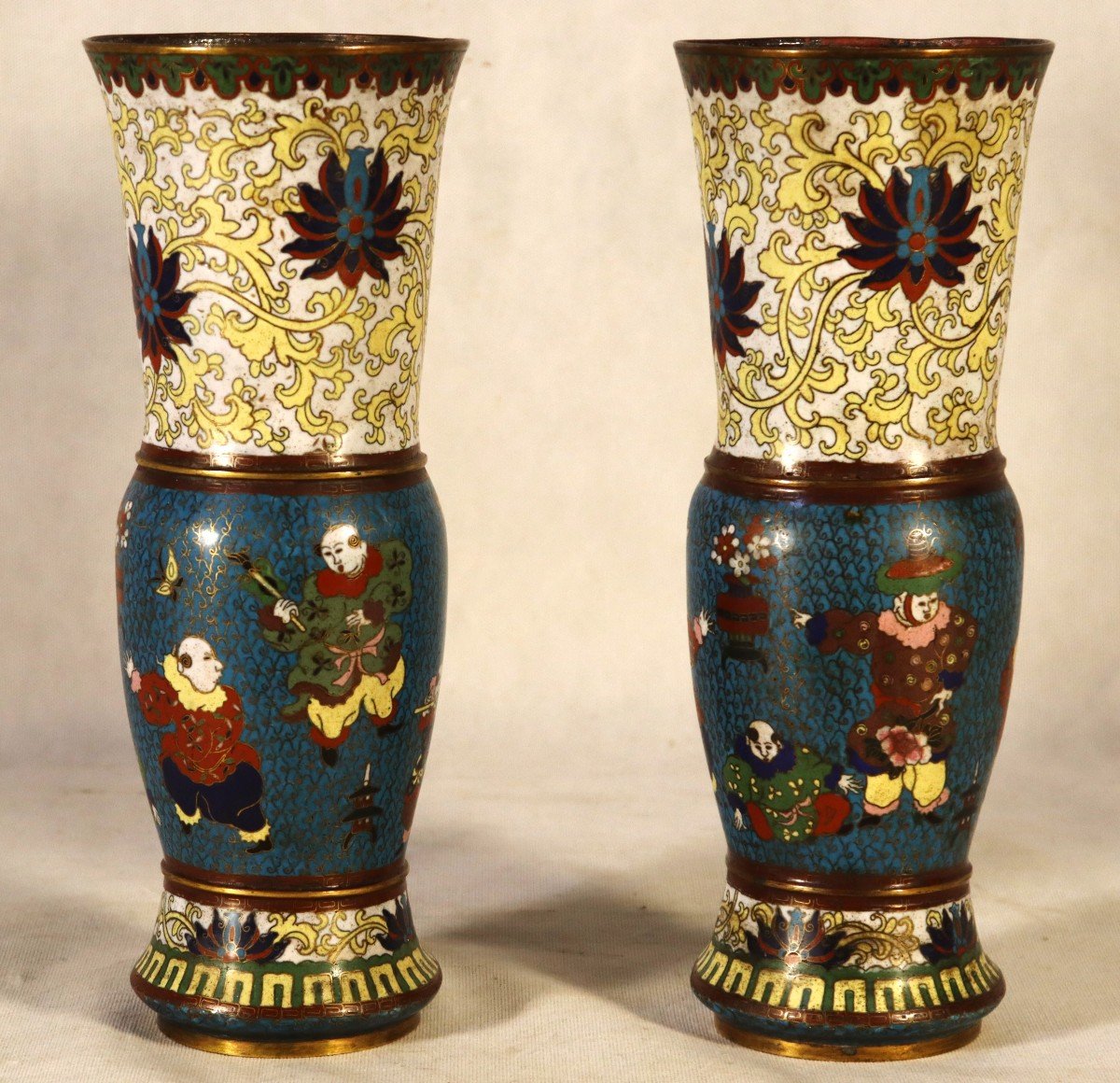This photograph features two virtually identical, intricately painted Chinese vases set against a gray background and floor. Each vase showcases an elaborate palette of colors, including shades of yellow, navy, dark blue, red, brown, black, and some green. Both vases feature a prominent blue band around their midsection where the main depictions are situated. 

On the left vase, two figures dressed in traditional Chinese costumes are vividly illustrated. One man wears an olive green tunic with a red collar, yellow pants, and red cuffed shoes, while the other wears a red shirt with a yellow collar, navy pants, and yellow cuffed shoes. Both men have white faces adorned with makeup and appear to be involved in some form of theatrical presentation, one holding what might be a sword or quill pen with a small pagoda at their feet. 

The right vase mirrors this but depicts two different men. One is standing, dressed in a brown tunic with a rosy collar, yellow trousers, and rose-trimmed boots, topped off with a green-rimmed hat with a brown center. The other man, seated and with a worried expression, wears a green tunic adorned with yellow flowers and red pants. Above them, a small pagoda decorated with vibrant flower blossoms in white, red, and brown is visible.

Both vases' tops exhibit coils of yellow and white flowers intertwined with black, green, brown, and red blossoms. The bases are trimmed with green and yellow, continuing the floral theme. These vases may be rendered in cloisonné, suggested by the texture and the outlining wires in the colorful designs, reminiscent of historic Chinese craftsmanship, possibly from periods like the Ming or Han Dynasty. The exaggerated features and jovial demeanor of the figures might suggest theatrical or clown-like representations, adding a layer of whimsy to the sophisticated artistry.